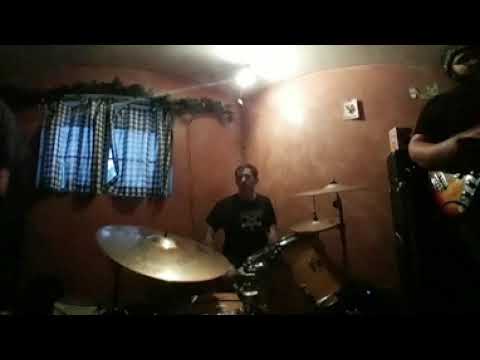In this indoor image, a man with dark hair is seated at a drum set, wearing a black t-shirt with an indistinct white logo. He is surrounded by orange and silver drums and a gold cymbal prominently positioned in front of him. His arms and drumsticks are not visible. The room appears aged and has a distinct atmosphere characterized by its darker tan, or perhaps pinkish walls. A white and blue checkered curtain covers an old window to the left of the drummer's head, and above it, a green, reef-like decoration hangs.

To the right of the drummer, partially in frame, stands another man wearing a black t-shirt and a beanie, playing a brown guitar. The room features a single overhead light and wooden dressers topped with white objects, adding to its vintage feel. The ceiling is white, and various elements like a white page with black text and a plant are tacked to the walls. The scene likely depicts a band practice session, with both musicians seemingly engaged in preparation.